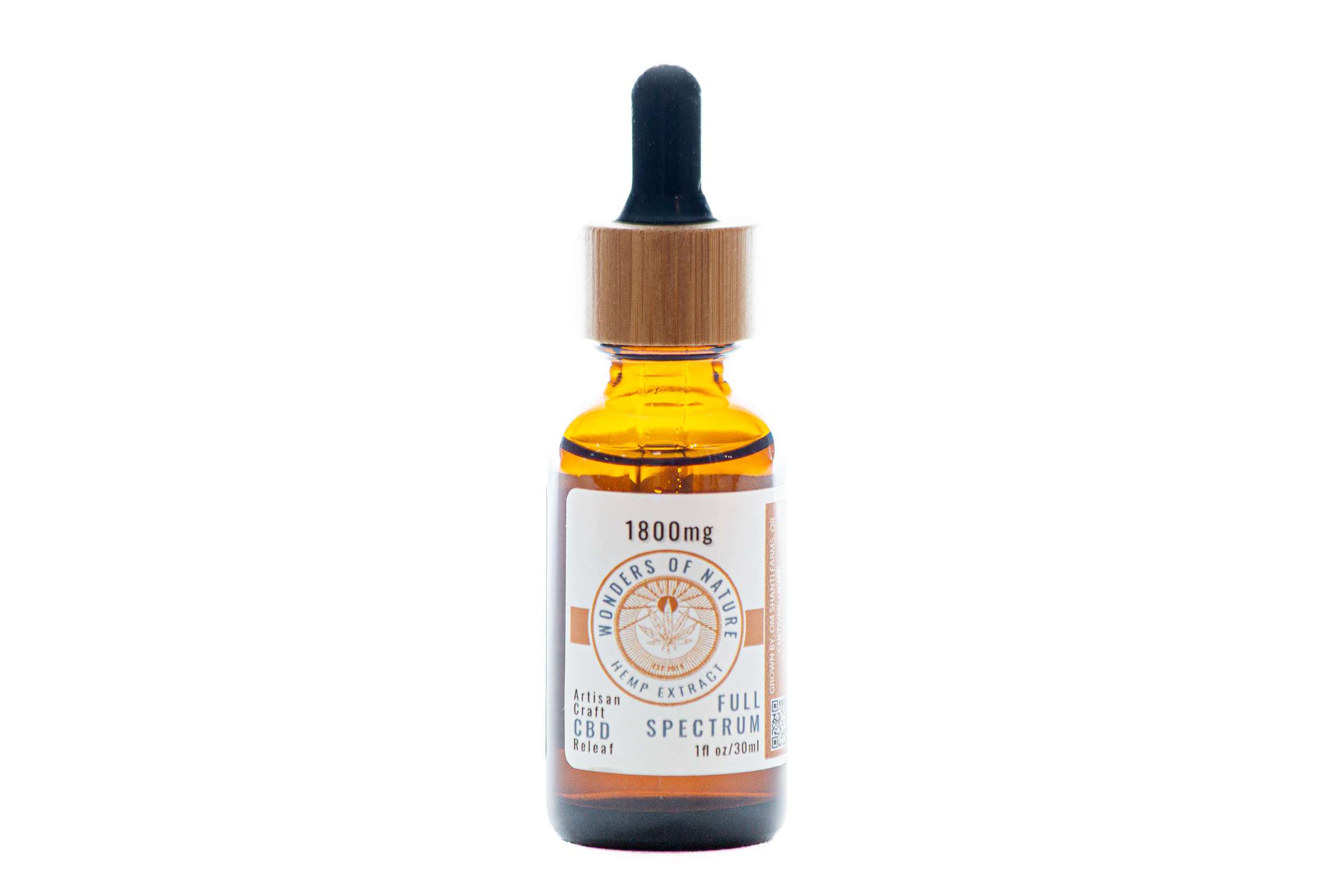This image showcases a brown glass dropper bottle prominently centered against a plain white background. The bottle contains a yellowish liquid, presumably a supplement. The dropper cap is wooden with a rubber black tip. The front label is predominantly white, featuring text and artwork arranged from top to bottom. It starts with "1800 MG," followed by "Wonders of Nature Hemp Extract" inside an orange circle with a leaf symbol. Below, it reads "Artisan Craft CBD Releaf," with the word "releaf" misspelled as "r-e-l-e-a-f," which undermines its credibility. Additionally, it mentions "Full-Spectrum 1 FL OZ / 30 ML," indicating it is a hemp extract product.